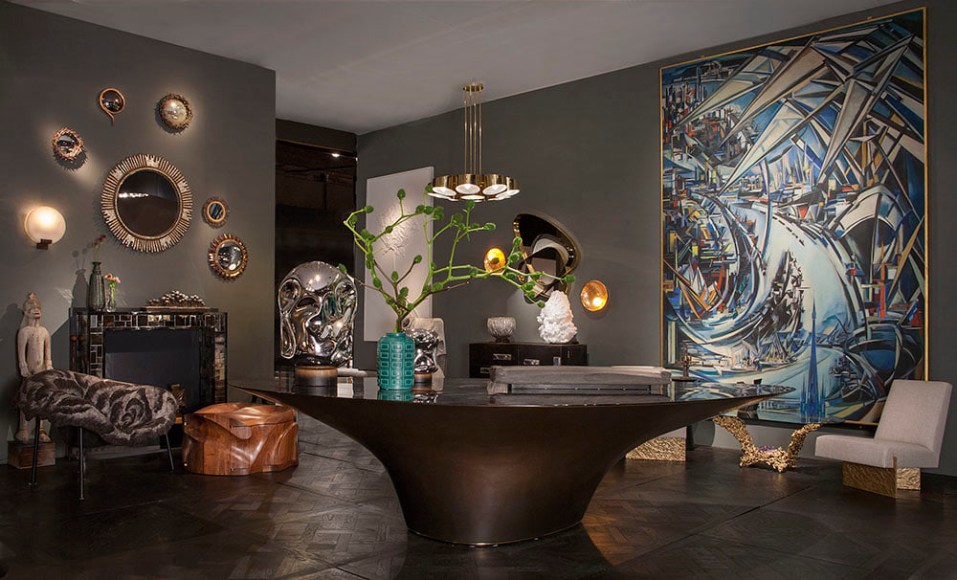The photograph depicts a sophisticated, modern living space with a distinctly artistic flair. The room features dark wood parquet flooring that complements the dark and moody ambience set by the gray, almost forest-green walls. At the heart of the space is a striking circular wood table with a glass top, adorned with a teal vase containing a green potted plant with bulbous leaves. Accompanying the plant are two chrome sculptures and a mysterious flat object, all of which contribute to the room's avant-garde aesthetic.

Against one wall hangs a large, colorful, abstract painting dominated by shades of blue and red, providing a vivid contrast to the muted walls. Below the painting, a white chair with a gold base is positioned next to a gold-and-glass side table. On an adjacent wall, a collection of gold-hued, circular mirrors and a sunburst mirror add a decorative touch above a modern glass fireplace.

In the left section of the room, a cozy setup includes a modern fur chair, a wooden ottoman, and a white chair draped with a fuzzy blanket. The setting is illuminated by a luxurious gold chandelier hanging from the ceiling. Overall, the space exudes elegance with its harmonious blend of modern art, plush seating, and rich, dark tones.